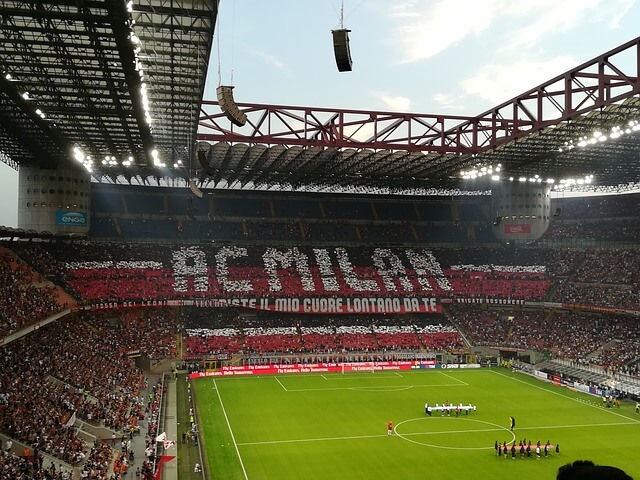This photograph captures an electric atmosphere inside a fully packed, open-air soccer stadium on a beautiful day with blue skies and scattered white clouds. Taken from the second tier of seats, the image shows a sweeping view across the field towards the opposite stands, highlighting the three levels of seating. On the pitch, both soccer teams are lined up, each holding their respective flags, signaling the beginning of the match. The fans on the opposite second tier are meticulously coordinated, spelling out "AC Milan" in massive white letters against a striking backdrop of red at the bottom, white in the center, and black at the top. The vibrant crowd in the stands is predominantly clad in these colors, showcasing their support for the home team, AC Milan. The stadium also features a retractable roof, which is almost fully open, allowing the sunlight to illuminate the green field lined with crisp white markings. In the center of the field, two individuals, one in a red shirt and the other in a black shirt, are standing within the center circle, adding to the anticipation of the game's kickoff.